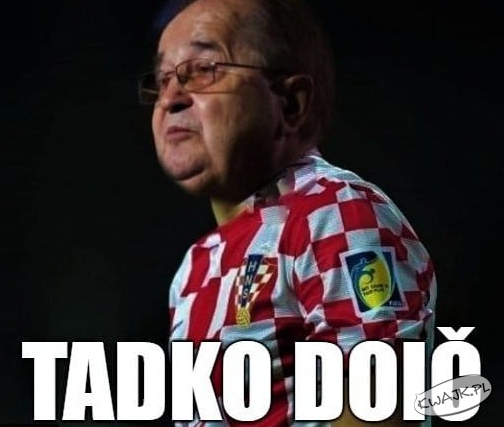An image depicts an older, heavyset man with a bald head and rimless, oval-shaped glasses. He is wearing a red and white checkered soccer jersey, identifying him possibly as a player or team member rather than an audience member. The jersey features an emblem over his left breast area that has "HNS" in white letters on a blue background, with a yellow soccer ball underneath. His left sleeve showcases a white outline image of a figure kicking a soccer ball, which is greenish with a blue border and yellow center, possibly containing illegible blue text. The dark, black background suggests the image might have been taken during a night event. Prominently at the bottom in large white letters is the name "Tadko Doyle," with the text "KWAJK.PL" appearing in gray over the letters "O" and "I."